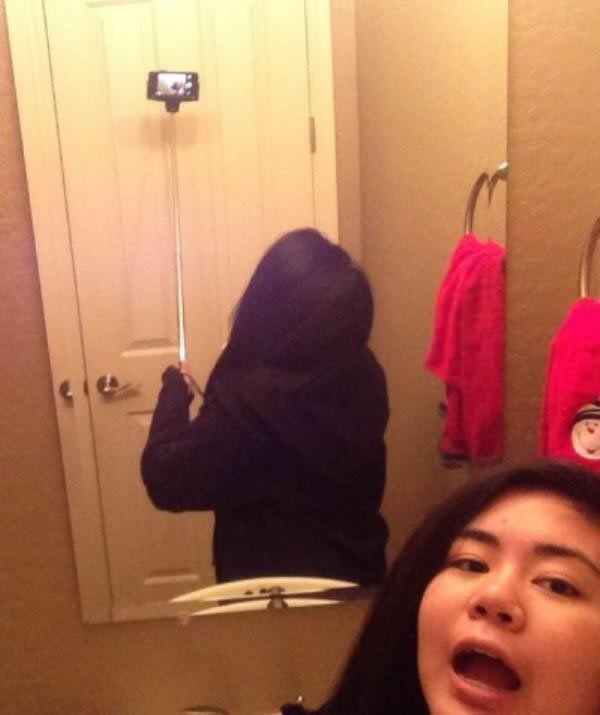A young woman, who appears to be Asian, is taking a selfie in her bathroom using a silver selfie stick. She is positioned in front of a rectangular mirror, with her back toward it, giving a clear view of both the front and back of her in the image. Her mouth is wide open, and her face is partially visible in the bottom right corner, showing brown eyes and possibly black hair hidden under a navy blue or black hoodie. 

In the reflection, the bathroom details are visible: a white door with a silver handle, a porcelain sink with a silver faucet, and a red snowman hand towel hanging on a towel loop. The hand towel features a white snowman with a carrot nose, adding a touch of color to the otherwise neutral bathroom setting. The overall scene captures the casual, light-hearted moment of the woman taking a selfie.